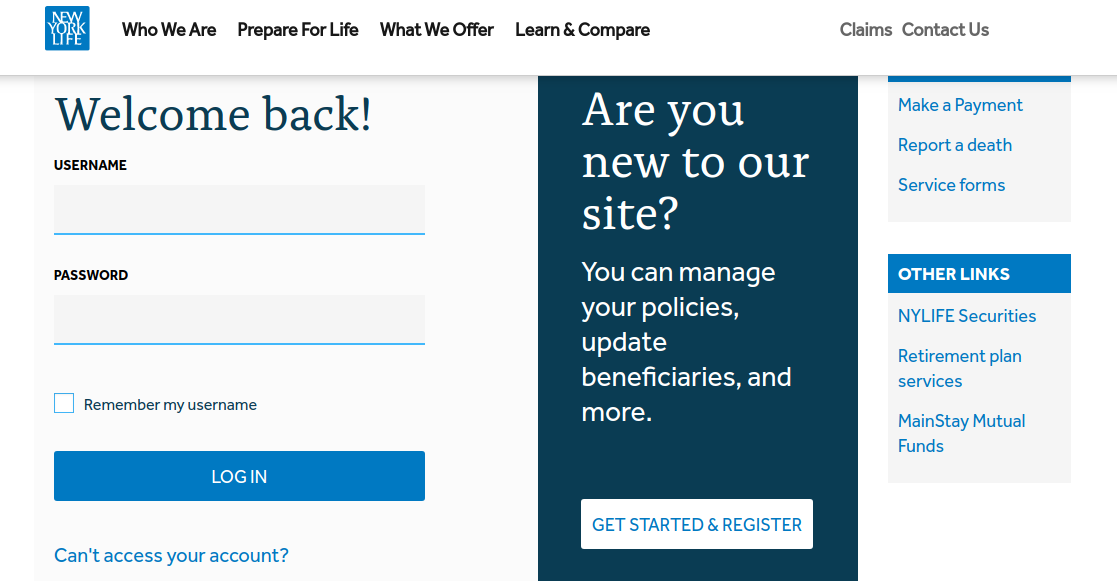The webpage for New York Life features a prominent blue square logo in the upper left corner, containing the words "New York Life" stacked vertically in white font. Adjacent to the logo at the top of the page is a nearly invisible white bar that sections off the navigation menu. The menu includes links sequentially titled: "Who We Are," "Prepare for Life," "What We Offer," "Learn and Compare," followed by "Claims" and "Contact Us" on the far right.

Immediately below the New York Life logo and the navigation menu, a large "Welcome Back!" greeting is displayed prominently. Below this greeting, the page has fields for user login: a "Username" field and a "Password" field, each represented as grayed-out rectangular boxes with blue lines at the bottom where users can enter their information. Accompanying these is a square checkbox labeled "Remember my username."

A rectangular blue "Log In" button spans the width equivalent to the input boxes below the login fields, featuring white text for the log-in prompt. Centrally located on the page, a prompt reads "Are you new to our site?" followed by an upright dark blue rectangle with white text offering assistance to new users.